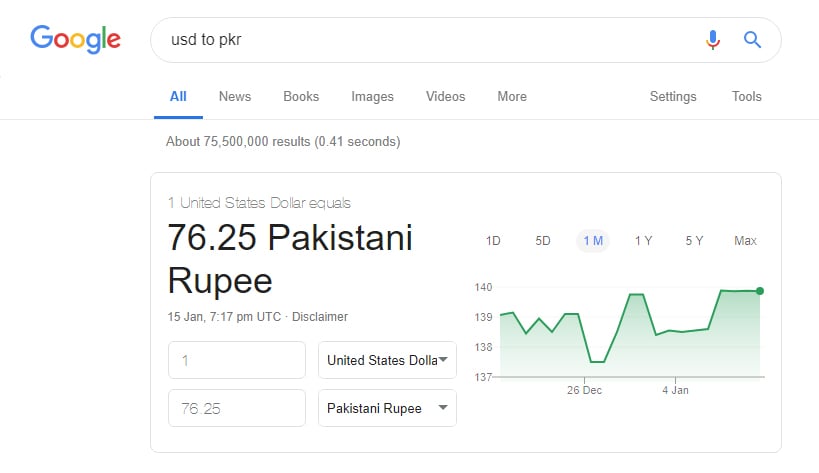A screenshot of a Google search results page is displayed. At the top of the page, "Google" is prominently positioned. Within the search bar, the query "USD to PKR" is clearly visible, indicating an inquiry about the exchange rate between the United States Dollar (USD) and the Pakistani Rupee (PKR).

Beneath the search bar, standard Google search categories such as "All," "News," "Books," "Images," "Videos," and "More" are listed. The current view is on the "All" category. The search has yielded approximately 75,500,000 results within 0.41 seconds, showcasing Google's rapid response capability.

Prominently displayed is the exchange rate stating that one United States Dollar (USD) is equivalent to 76.25 Pakistani Rupees (PKR). For illustrative purposes, this can be approximated to 75 Rupees per Dollar, suggesting that the Dollar holds about 25% more value than the Rupee.

Additionally, the timestamp indicates the rate was retrieved on January 15th at 7:17 p.m. UTC time. Below the exchange rate are drop-down menus that allow for the conversion of USD to various other currencies, such as Francs, Pesos, and others.